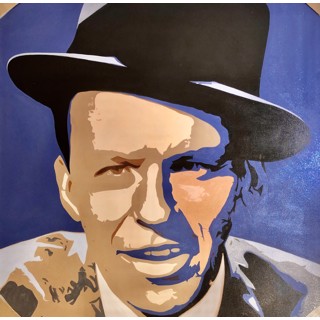The image features an abstract, yet discernible painting of a man who resembles Frank Sinatra. His slightly tanned Caucasian face, highlighted in varying shades of beige, dark beige, and light beige, stands out against a predominantly blue background. The man's right side is enveloped in blue shadows, accentuating his eye, nose, lips, chin, and even his ear in a cooler hue. He sports a black top hat, tipped slightly to the right, though the top part of the hat extends beyond the frame. He has black hair peeking from beneath the hat. His attire consists of a beige or tan coat with a white dress shirt underneath. The background is predominantly blue, interspersed with purple tones and small brown triangles in the upper corners. The composition extends from the top of his hat to just below his shoulders. The man is captured with an open-mouthed smile, revealing his upper teeth.